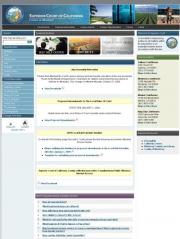This image showcases a formal website that appears to be designed similarly to a government portal. On the left side of the webpage, there is a circular emblem, possibly representing "Lawrence Court" or something similar. The top of the page features a blue header with the website's name. To the right of the header, there are four distinct images: one depicting a tropical area, another that appears to be an aquarium tank, a third showing fields on a farm, and the last one of a beach. Beneath the header are two navigation bars: one with clickable sections presumably leading to different site areas, and a drop-down menu on the left offering various links. The main body of the webpage contains a large amount of illegible text. On the right-hand side, there is a section that likely displays contact information for individuals holding various positions within the organization.